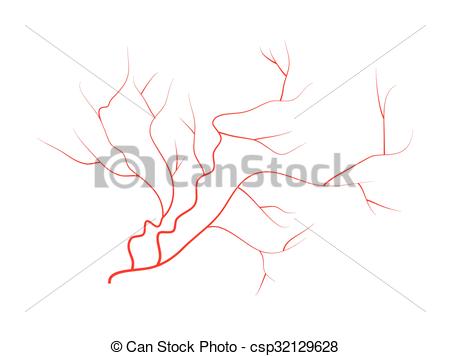This is a detailed drawn illustration of a complex network of red arteries, prominently stemming from a main branch that bifurcates into five smaller offshoots, which in turn further subdivide, creating a tangled web of blood vessels. The background is dominated by a light gray, fragmented X-like structure, contributing a sense of depth, and interspersed by thin, wispy red branches evocative of the blood vessels. Across the image, there is a faint overlay of a camera icon and the text "Can Stock," emphasizing its nature as a stock photo. The colors utilized in the image include deep red for the arteries, contrasted against black and various shades of gray and white in the background. At the bottom, the text reads "Copyright Can Stock Photo CSP 32129628," indicating the need for proper permissions to use the image without watermarks. The layout is horizontal, with the text centrally aligned, highlighting the arteries sprawling in various directions.